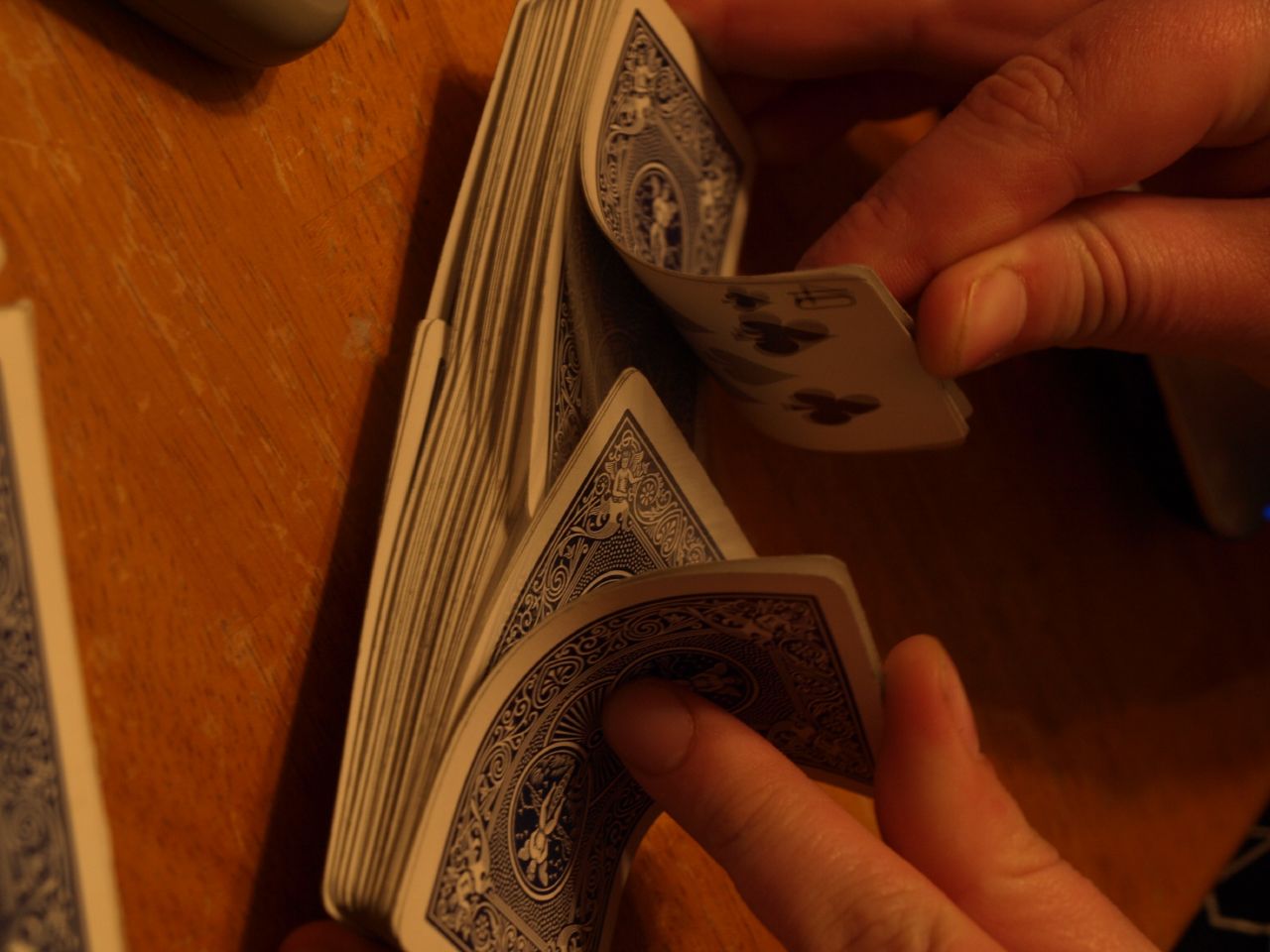In this image, we see a close-up of a person shuffling a deck of cards. The focus is on the intricately designed, dark blue cards with white patterns and edges. At the bottom of the image, a small portion of one card is visible, showing a dark blue backside with detailed white designs and a white border. The cards are placed on a light brown, golden-colored table that extends throughout the image.

To the bottom left corner, a gray object casts a shadow, hinting at an unseen item just outside the frame. Above this, the cards are captured in mid-shuffle, indicating a dynamic motion. One of the cards in the deck, identified as the ten of clubs, is slightly bent upwards due to the shuffling action.

Emerging from the top edge of the image are two hands actively engaged in the shuffling process. The left hand shows three fingers, while the right hand shows two, both gripping the tops of the cards firmly. The table surface continues beyond the hands, completing the background of this detailed and dynamic scene.